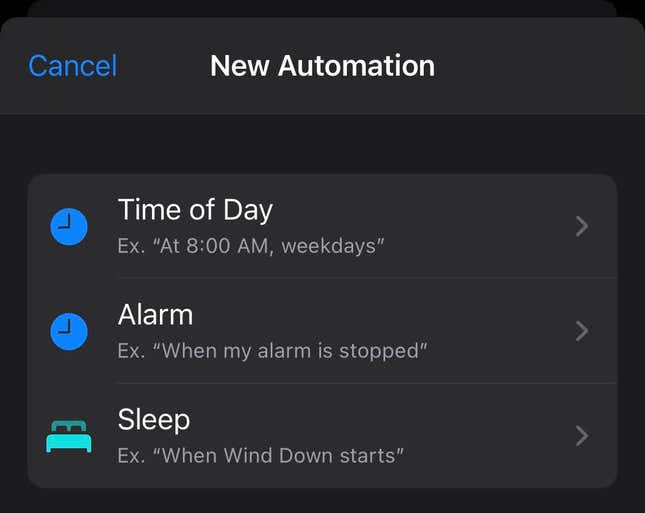The image depicts a horizontal rectangular screen featuring a user interface, likely from a mobile device. At the top left corner, the word "Cancel" appears in blue text. Centered at the top is the title "New Automation," displayed in white.

Below the title are several sections, each denoted with specific icons and text descriptions:

1. **Time of Day:**
   - Icon: Blue clock.
   - Description: "At 8 a.m., Weekdays."
   - Arrow: Right arrow symbol.

2. **Alarm:**
   - Icon: Blue clock.
   - Description: "When my alarm is stopped."
   - Arrow: Right arrow symbol.

3. **Sleep:**
   - Icon: Green bed.
   - Description: "When Wind Down starts."
   - Arrow: Right arrow symbol.

The text "Wind Down" is capitalized, whereas "starts" is not. The screen features a color palette of blue, green, white, gray, and black. There is no explicit identification of the device, but the layout suggests it is likely a smartphone interface.